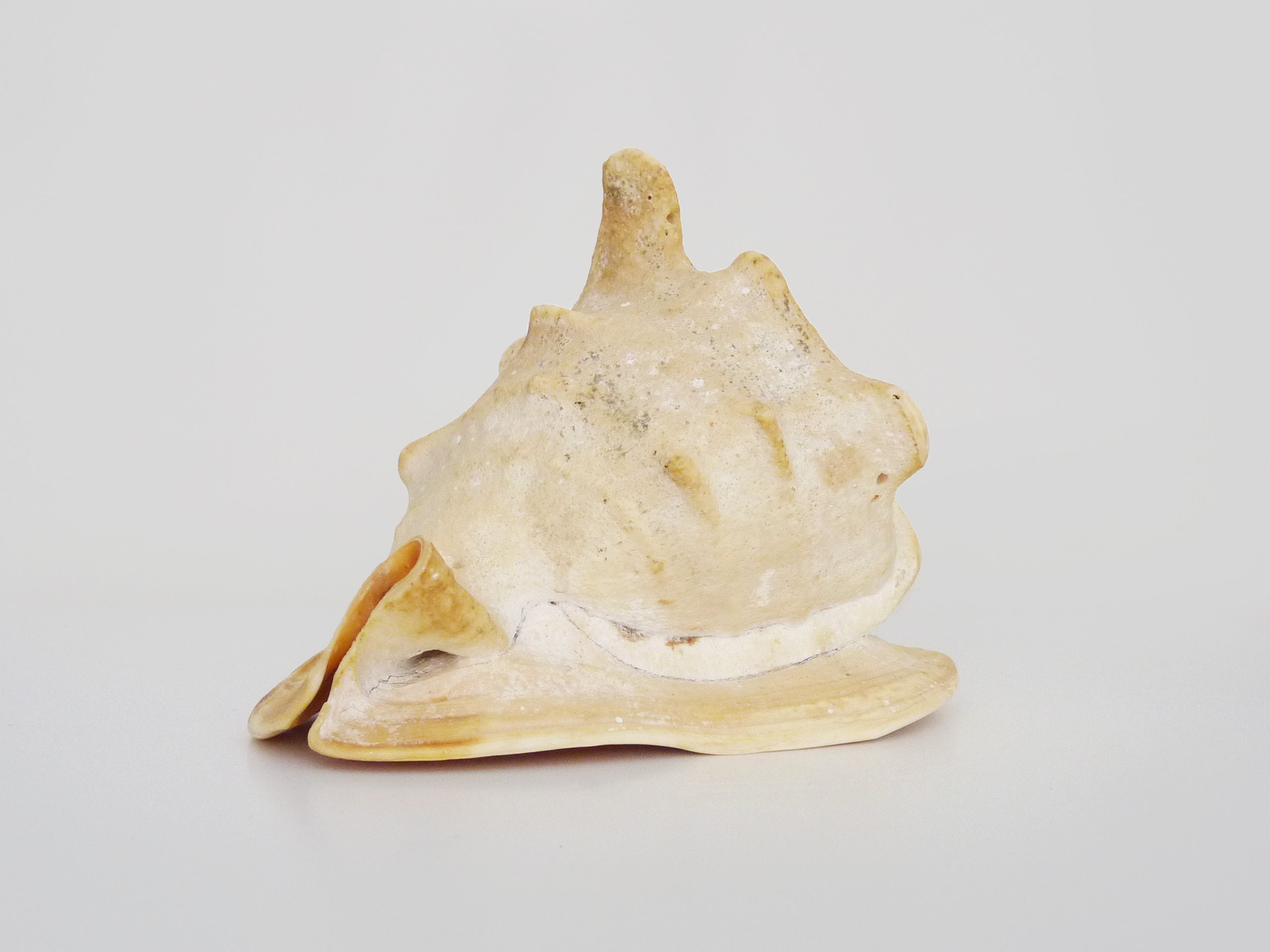This is a color photograph of a seashell, centered against a solid gray background. The shell itself is predominantly pale yellow with hues of light brown and sand. It features a significant amount of detailed texture, including bumps on its exterior and a prominent, horn-like protrusion at the top. The upper part of the shell appears to serve as a protective covering, while underneath, two flatter shell sections extend and seem to form part of the main body. The raised portions of the shell display a rust color, particularly evident where the shell curves upwards to an opening on the left side. The interior of the shell is a darker rust shade. The shape and substantial size of the shell suggest it could have been a suitable home for marine creatures like a conch or a hermit crab. The image is sharply focused on showcasing the intricate textures and colors of the seashell, making it the sole subject of the composition.